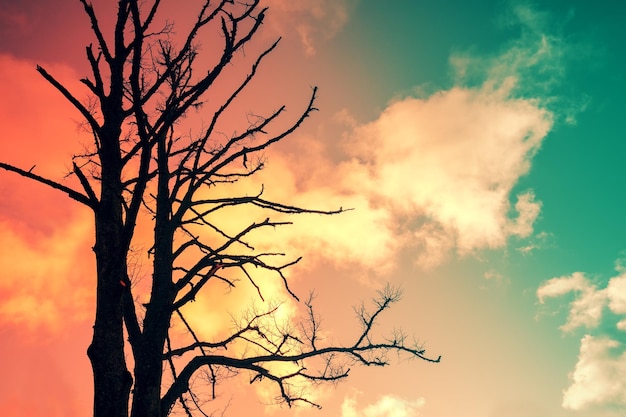This captivating outdoor photograph captures a stunning sunrise or sunset with a sky that transitions through various hues. Dominating the scene is a tree in shadow, rendered in silhouette due to the lighting and angle of the camera. The tree, with its many branches but devoid of leaves, stands prominently in the foreground. It appears alongside another similarly bare tree, suggesting either a pair of trees or a single tree with a split trunk.

The sky is a tapestry of colors, with a vast majority covered in warm reddish-orange, peach, and gold tones blending seamlessly. The left side features a particularly striking palette, with deep orange and yellow shades interspersed with patches of purple. Puffy white clouds float below the peach-hued sky. On the right side, the photograph transitions into a seafoam green and turquoise blue sky, speckled with additional white clouds. This careful interplay of colors and the stark, shadowed profile of the leafless trees creates a compelling contrast, enhancing the beauty and depth of the scene.